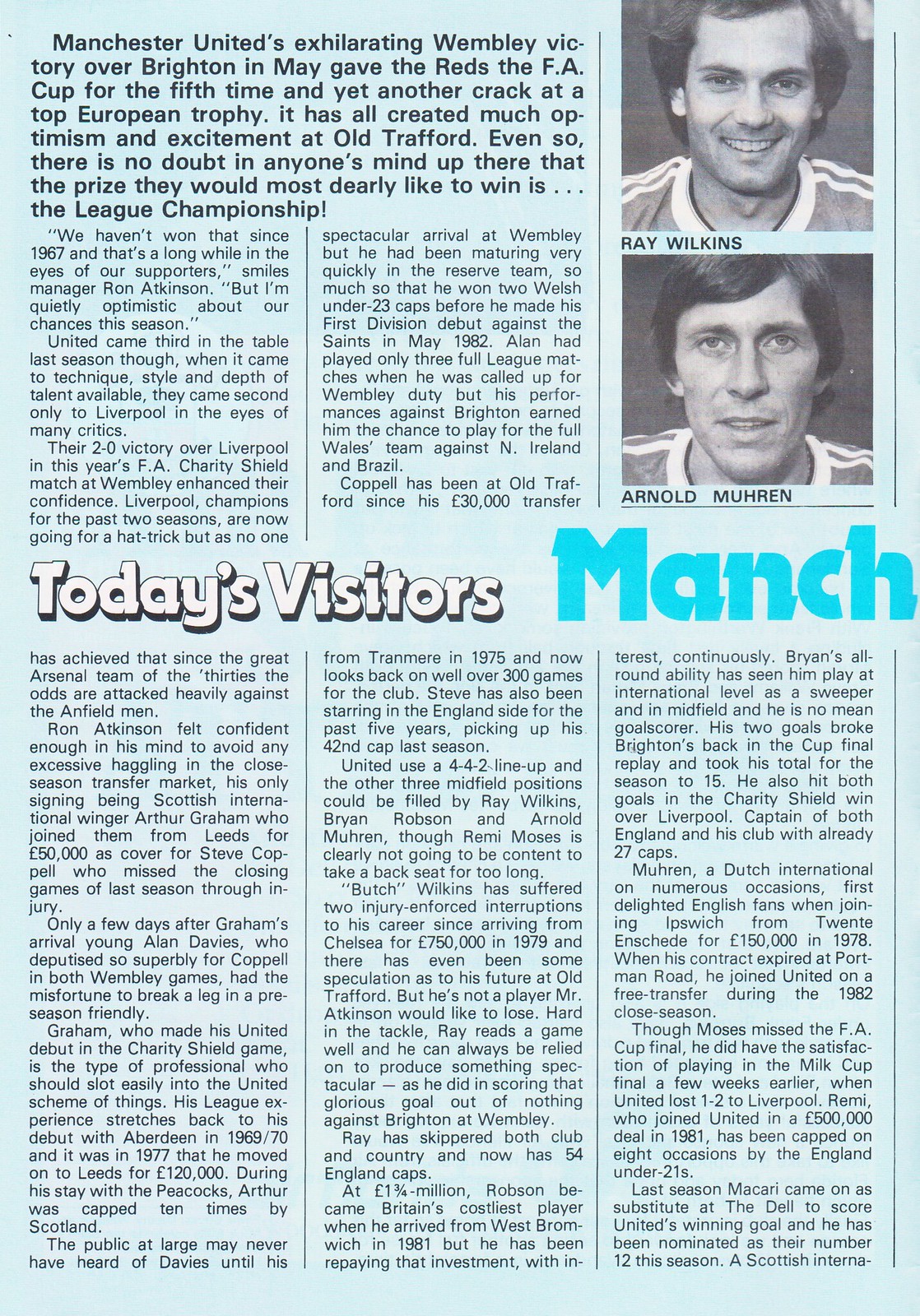The image depicts a light blue page from an old newspaper or booklet, containing a detailed article about Manchester United's exhilarating Wembley victory over Brighton in May. This triumph awarded the Reds the FA Cup for the fifth time, rekindling hopes for a top European trophy and generating optimism at Old Trafford. Central to the page are two black and white photographs in the top right corner: one of Ray Wilkins and another of Arnold Muren, both smiling for the camera. The text emphasizes that despite their FA Cup win, manager Ron Atkinson and supporters are most eager to clinch the League Championship, a title they haven't secured since 1967. The article mentions Manchester United's third-place finish in the league last season, noting their superior technique, style, and depth of talent, second only to Liverpool. Their confidence was further bolstered by a 2-0 victory over Liverpool in the FA Charity Shield match at Wembley. A prominent headline in the middle of the text reads, "Today's Visitors Manch," indicating the context of the article within the broader publication.